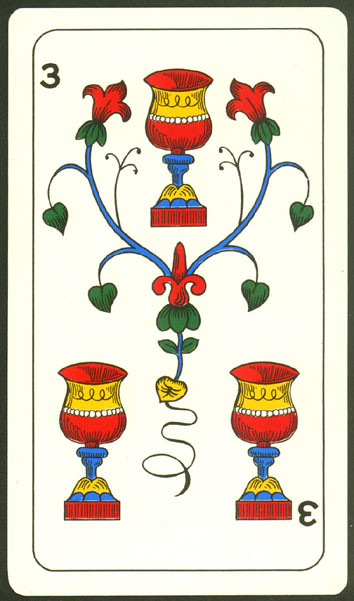This image showcases a single, intricately designed card with an elegant yet antiquated appearance. The card features a thin black border surrounding an off-white, slightly dingy background. In the top left corner of the card, there is a prominently displayed black number "3." 

The card is adorned with multiple detailed elements, including two opulent chalices depicted in gold, red, white, blue, and yellow hues. Another upside-down black number "3" is positioned at the bottom of the card, maintaining the card's symmetry.

The center of the card is dominated by a complex floral design. This design includes a yellow leaf, several green leaves, and a striking red object with two horn-like projections, alongside an additional object protruding between them. Intertwined blue vines permeate the design, with green and red floral leaves adorning the topmost portions.

Topping off the card's intricate imagery, another chalice—similarly adorned in yellow, gold, red, white, and blue—is placed at the uppermost section. The card's detailed artwork and vibrant color scheme are the sole features, making it a fascinating and visually rich example of its kind.